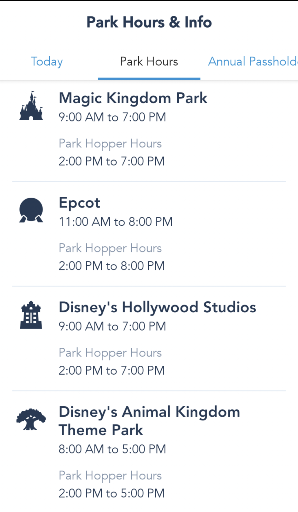A mobile phone displays a detailed page titled "Park Hours and Info," featuring a header with a black line above the text. Below the header are three columns labeled "Today," "Park Hours," and "Annual Pass Holder," though the third label appears cut off. The background of these columns has a blue line beneath "Park Hours."

Following the header, the page lists various theme parks and their operating hours:
1. **Magic Kingdom Park** - Represented by a castle icon, showing specific operating hours.
2. **Epcot** - Illustrated with a globe and hand icon, detailing its own set of hours.
3. **Disney Hollywood Studios** - Denoted by a classic arched doorway icon, along with its operating times.
4. **Disney's Animal Kingdom Theme Park** - Marked by a tree icon, accompanied by its hours of operation.

Additionally, each park's section lists "Park Hopper Hours," which are different from the standard park hours provided. The significance of "Park Hopper Hours" is not explained in the image.